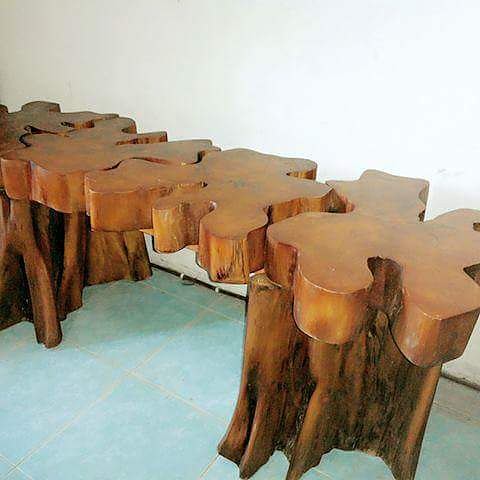The image features a beautifully carved and ornate piece of furniture, most likely a coffee table or bench, though its exact size is hard to discern from the given perspective. The table's top is crafted from four substantial, thick, medium brown-orange hued interlaced wood slices, meticulously fitted together like a puzzle. There are small gaps between the slices, with one noticeable gap on the right, possibly due to the photo's angle. The surface is polished and finely sanded, indicating a high level of craftsmanship. The table is supported by two rough sections of tree trunks, acting as legs, which are positioned on the far left and far right sides. These trunks retain their natural ridges and indentations, contributing to the piece's rustic charm. The table stands on a pale aqua tile floor with a white pattern and is set against a white wall. The entire composition is captured within a square frame, presented at a slight diagonal, enhancing the unique and abstract aesthetic of this wooden furniture.